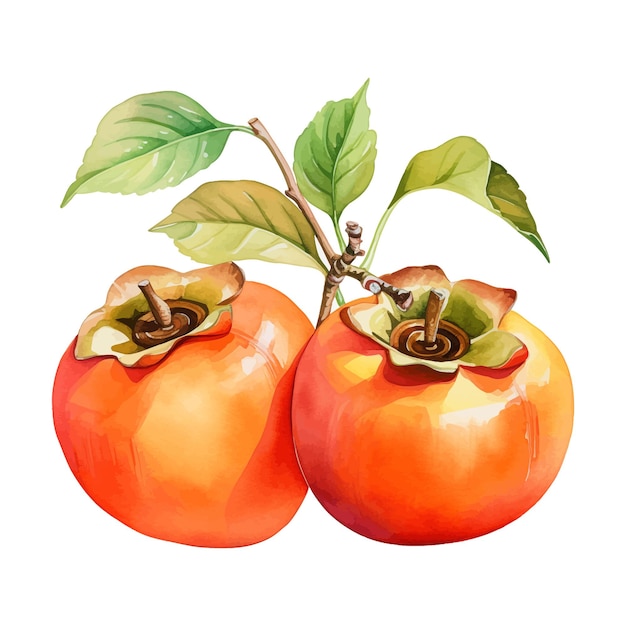In the image, there is a detailed illustration of two closely positioned fruits that appear to be tomatoes, depicted in a cartoon-like, clip-art style. These tomatoes are a vibrant mix of red and orange, with shiny surfaces highlighted by reflections of light. The fruit on the left is nearly perfectly round, while the tomato on the right tapers to a point at the bottom, resembling the shape of a strawberry and has a small droplet of liquid on its side. Both fruits have green sepals crowning their tops, indicating where they were once connected to their branch. Behind the tomatoes, a small brown branch holds four green leaves, adding a touch of realism and context to the illustration. The background of the image is a plain white, emphasizing the bright colors and glossy textures of the depicted fruits.